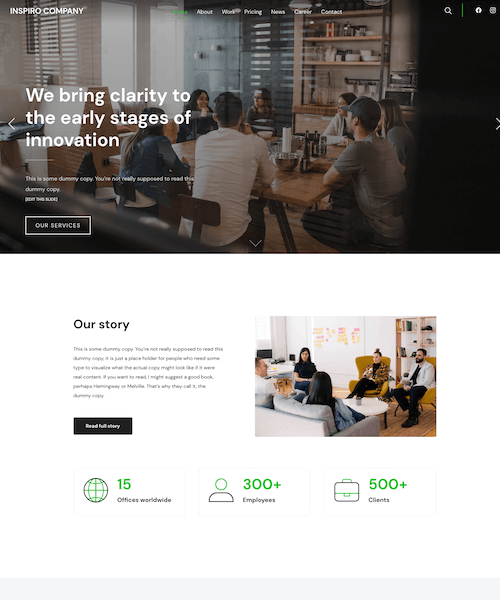Here is a detailed and cleaned-up caption for the image described:

### Inspiro Company Homepage Screenshot

The top half of the image showcases a professional photograph featuring a group of seven people seated around a modern, large table. The setting appears to be inside a chic, contemporary residence or possibly a high-end restaurant. The overall lighting is slightly dim, creating a cozy yet professional ambiance. Superimposed on this photograph, in white font, is the Inspiro Company logo positioned at the top left corner. To the right of the logo, a navigation bar displays links to "About," "Work," "Pricing," "News," "Career," and "Contact,” accompanied by a search icon on the far right.

Prominently displayed in large white text on the left side is the company’s tagline: "We bring clarity to the early stages of innovation." Beneath this, in smaller white text, is placeholder text, commonly known as dummy copy, not intended for actual reading. Additionally, there is a rectangular button outlined in white labeled "Our Services."

The bottom half of the image features a white background with the title "Our Story" and more dummy copy. Adjacent to this title, a black button urges viewers to "Read Full Story."

To the right of this section is another image depicting five individuals: two seated on a couch and three on chairs, with a coffee table centered between them. Below this image, green text highlights the company’s global presence: "15 offices worldwide," "300+ employees," and "500+ clients.”

This detailed caption provides an accurate and comprehensive description of the content and layout of the Inspiro Company’s homepage screen.